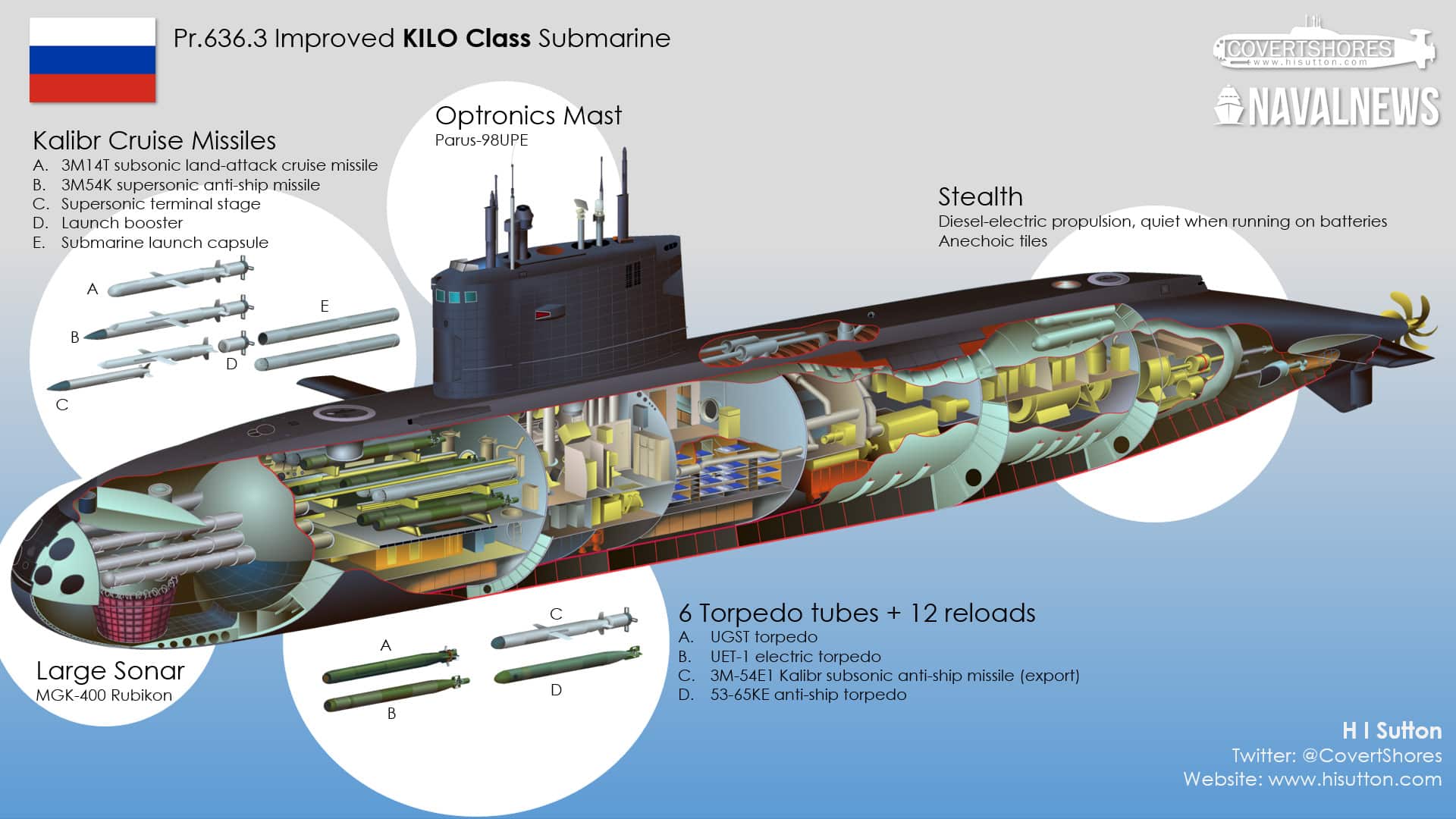This detailed diagram, sourced from "Naval News" magazine, features the PR 636.3 Improved Kilo Class Submarine. In the upper left corner, a flag with three bands of white, blue, and red colors is visible, along with the label "PR 636.3 Improved Kilo Class Submarine" and the titles "Covert Shores" and "Naval News". The right corner details the stealth capabilities, including diesel-electric propulsion and quiet operation on batteries, with an anechoic tiles coating.

The submarine's cross-sectional view showcases its intricate interior. The top section is annotated with labeled Caliber Cruise Missiles from A to E, and the "Optronics Mast" positioned prominently. Beneath, the large sonar system is highlighted near the submarine's nose. The diagram details six torpedo tubes with twelve reloads, along with A to D labeled torpedoes bays. The bottom section, colored blue to simulate water, contains additional labeling and technical details.

White lettering on the right side notes the name H.I. Sutton, with associated Twitter handle @CovertShores and website www.hisutton.com. This comprehensive illustration provides a thorough insight into the structural and operational components of the submarine, blending technical and visual elements seamlessly.